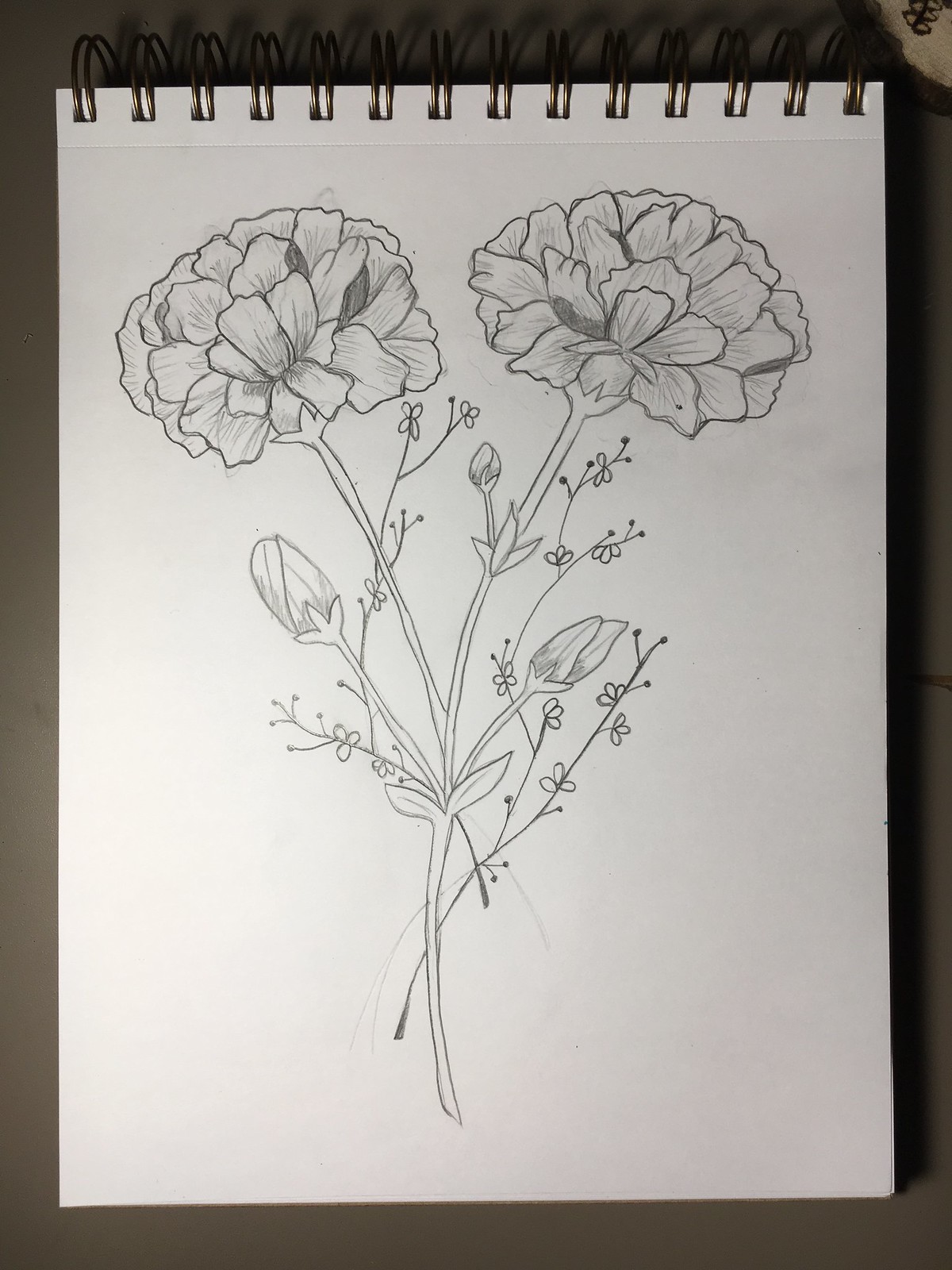In this image, we see a detailed pencil sketch on an A4 portrait orientation drawing pad, resting on a gray table with a black background. The notebook has spiral metal rings at the top. The sketch features two prominent, rose-like flowers in full bloom, interconnected at their stems. Surrounding these blossoms are several smaller buds—two medium-sized and one very small—that have not yet opened. Thin branches extend from the stems, adorned with tiny petals and leaves. The paper is white and unlined, indicating a sheet meant specifically for drawing. Visible pencil marks hint at some erasing and reworking, adding a textured shadowing effect to the petals. Overall, the sketch is well-drawn, capturing fine details and demonstrating careful shading, yet it remains a monochromatic pencil illustration without color or text.